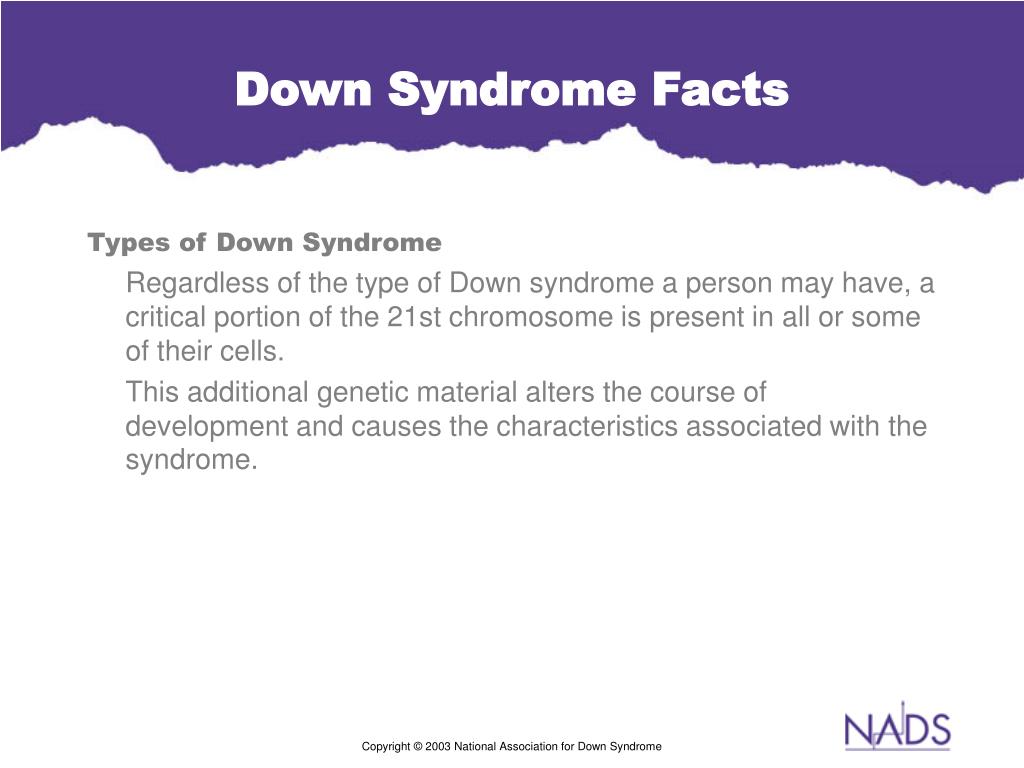Screenshot of a computer screen displaying a webpage on Down Syndrome. The top section features a purple border with a frayed, torn-like design at the bottom. In the center of the border, bold white text reads "Down Syndrome Facts." Below, against a white background, the heading "Types of Down Syndrome" appears in gray in the upper left corner. The text explains that regardless of the type of Down Syndrome, a critical portion of the 21st chromosome is present in all or some cells, causing the developmental changes and characteristics associated with the syndrome. Towards the bottom of the white background is a note in small print: "Copyright 2003, National Association for Down Syndrome," with a circled "C" symbol next to "copyright." In the bottom right corner, "NADS" is written in purple and underlined with a purple line. The letter "A" features a distinct design with a line starting from the bottom left, crossing through the middle, and extending to the top right.